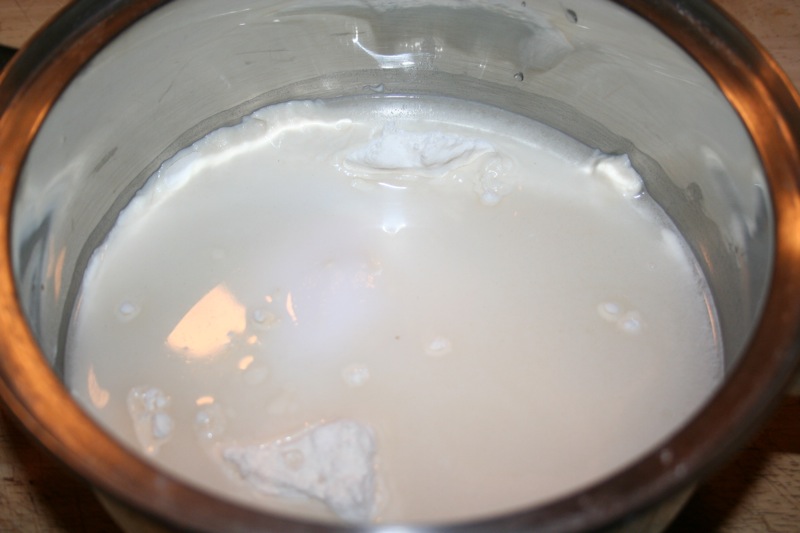This detailed rectangular photograph captures a round pot or glass bowl with a stainless steel interior, set against a barely visible tan countertop, likely made of a material such as granite or wood. The pot features a metallic frame with a stainless steel rim that glows with a silvery sheen, possibly reflecting the light source, and carries a hint of a copper color due to the lighting. Inside the pot, there is a white, sticky, and chunky substance that resembles milk mixed with possibly flour or chunks of cream cheese, suggesting that someone might be in the process of creating a roux. The overall scene gives prominence to the reflective metal and the creamy contents within the pot, creating a visually intriguing and culinary-focused image.